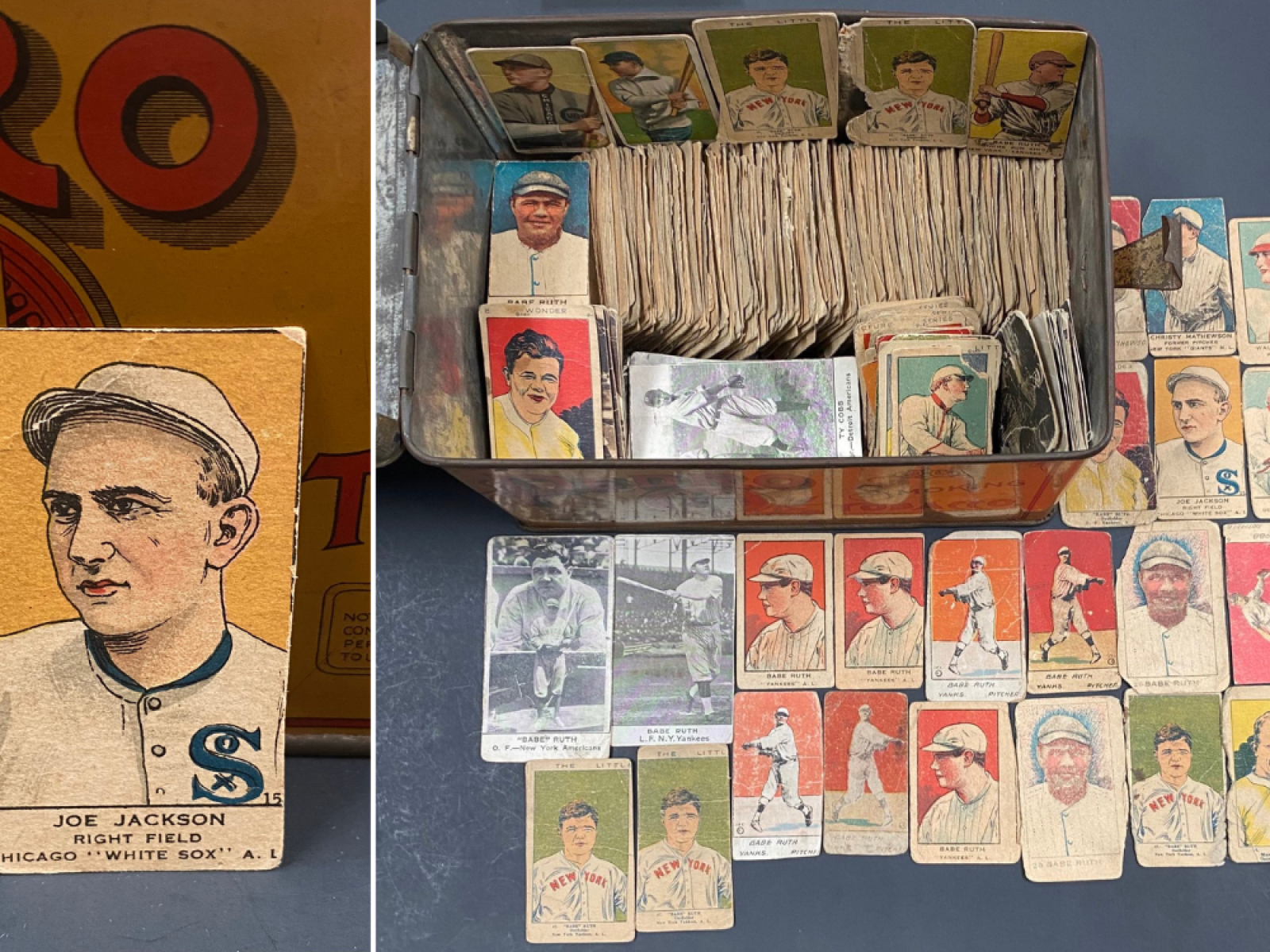The image consists of two separate photographs. The left side showcases a close-up of an old baseball trading card of Joe Jackson from the Chicago White Sox, labeled "Rightfield Chicago White Sox." The card features a cartoon of Jackson, who is clad in a white cap and a white jersey accented with blue, displaying a large blue "S" on the right and three buttons down the front. On the right side, there is a photograph of a metal bin brimming with numerous worn baseball cards. Many of these cards are spread out on the table in front of the bin, arranged side by side, showcasing a mix of black and white and colorful cards with vibrant backgrounds in hues of yellow, orange, red, green, and blue. Some cards are duplicates, and many are visibly aged, with tears, wrinkles, and fading colors, giving a glimpse into an extensive and well-used collection of vintage baseball memorabilia.